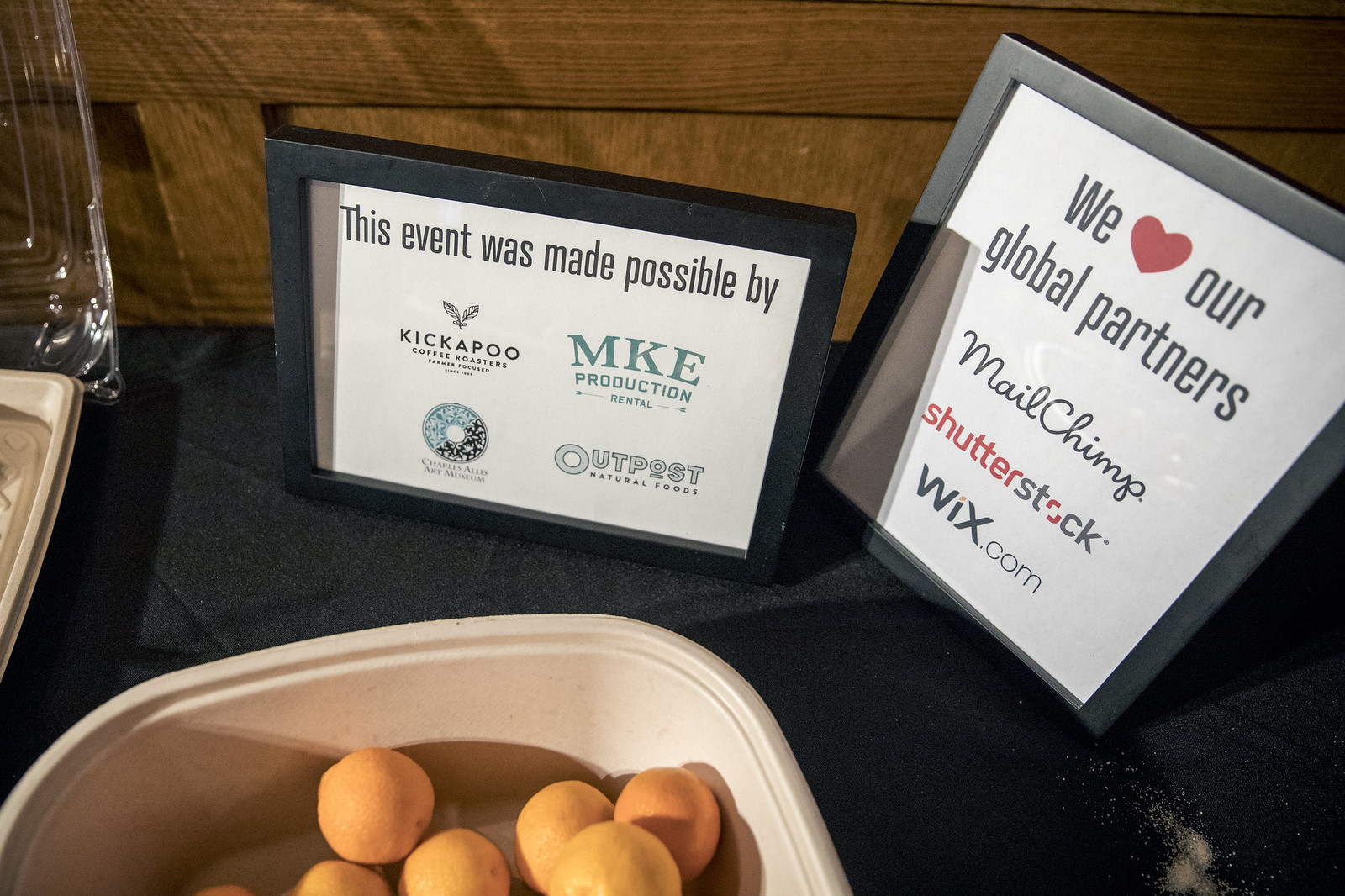This indoor image features a wooden wall backdrop and a table draped with a black tablecloth. Prominently displayed at the center are two distinct frames. The black frame on the left highlights event sponsors, stating, "This event was made possible by," followed by logos for Kickapoo Coffee Roasters with intertwined leaves, MKE Production Rental in green, and Outpost Natural Foods in light gray and black. Adjacent to this is a vertically oriented gray frame, inscribed with "We ❤️ Our Global Partners" in black text, listing partners MailChimp in cursive, Shutterstock with "Shutter" in red and "stock" in gray (with an orange 'O'), and Wix.com in bold black. In front of these frames is a tan, rounded square container filled with approximately six visible oranges or clementines, adding a vibrant pop of color. The setting suggests an event space, with a variety of objects including trays partially visible to the side.